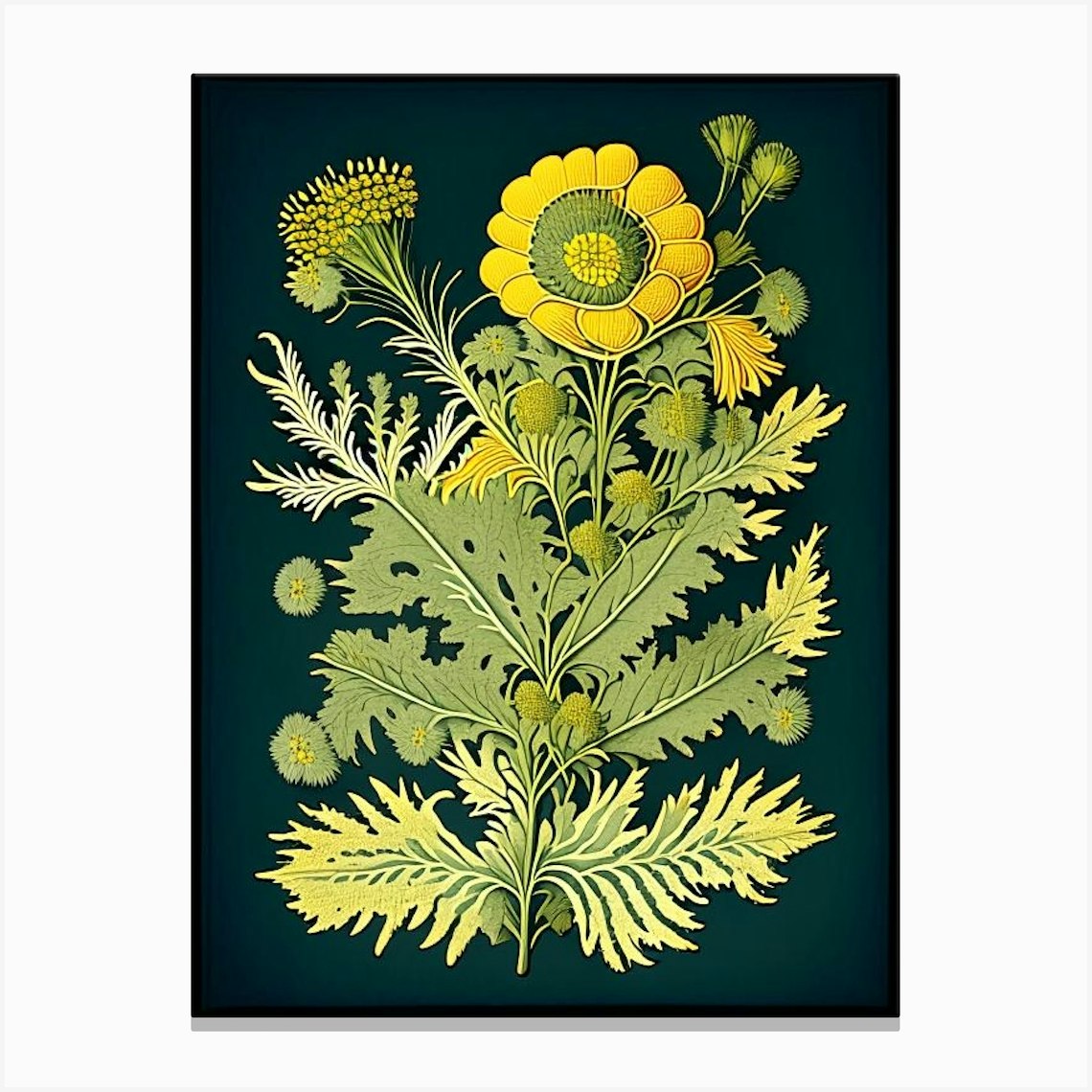This is a detailed image of an artistically rendered green flower, set against a rich, dark green backdrop. The flower, prominently stretching through most of the picture, features several paired green leaves protruding in sets of two, four, and six. At the top, the flower culminates in a vibrant, fully bloomed dandelion-style blossom with bright yellow petals encircling a green and yellow center. Surrounding the central flower are smaller blooms and buds in varying states of growth, adding depth and texture to the scene. The piece appears to be a combination of stitches, embroidery, and possibly paint, showcasing delicate craftsmanship. The entire composition is framed in a tall rectangular format, highlighting the intricate details and the beauty of the flower's progression from stem to bloom.